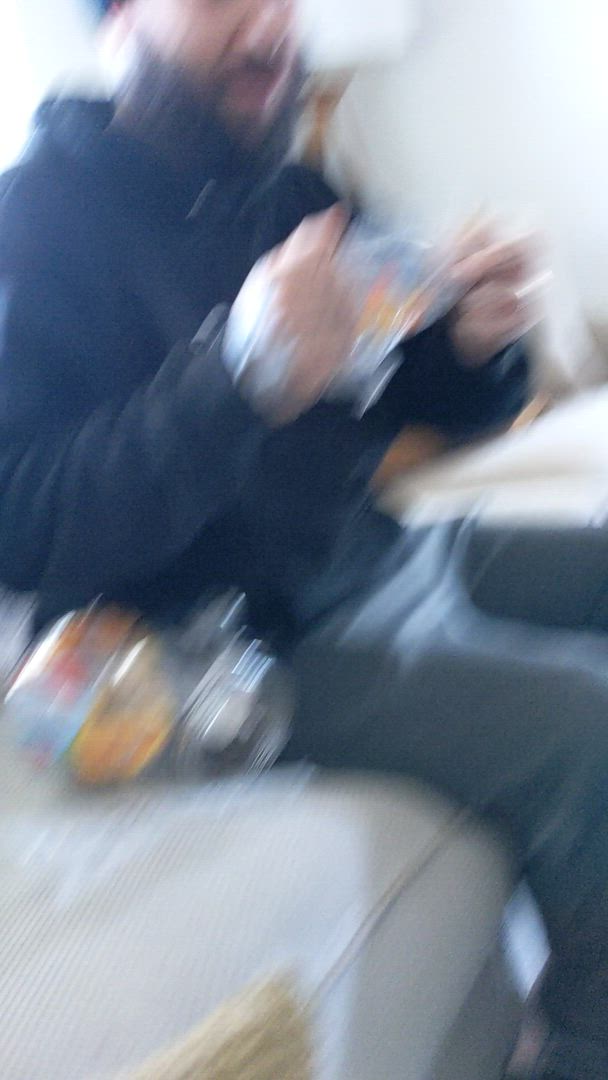In this extremely blurry indoor photograph, a man is seen seated on a white couch against a backdrop of white walls. He is dressed in gray pants and a black hoodie, accessorized with a silver watch on his wrist. The man's features include a prominent black beard. Although the image quality is poor, he appears to be holding a colorful object encased in a clear package. On the couch beside him, two identical clear packages containing colorful items are also visible, hinting at some intriguing activity or collection.